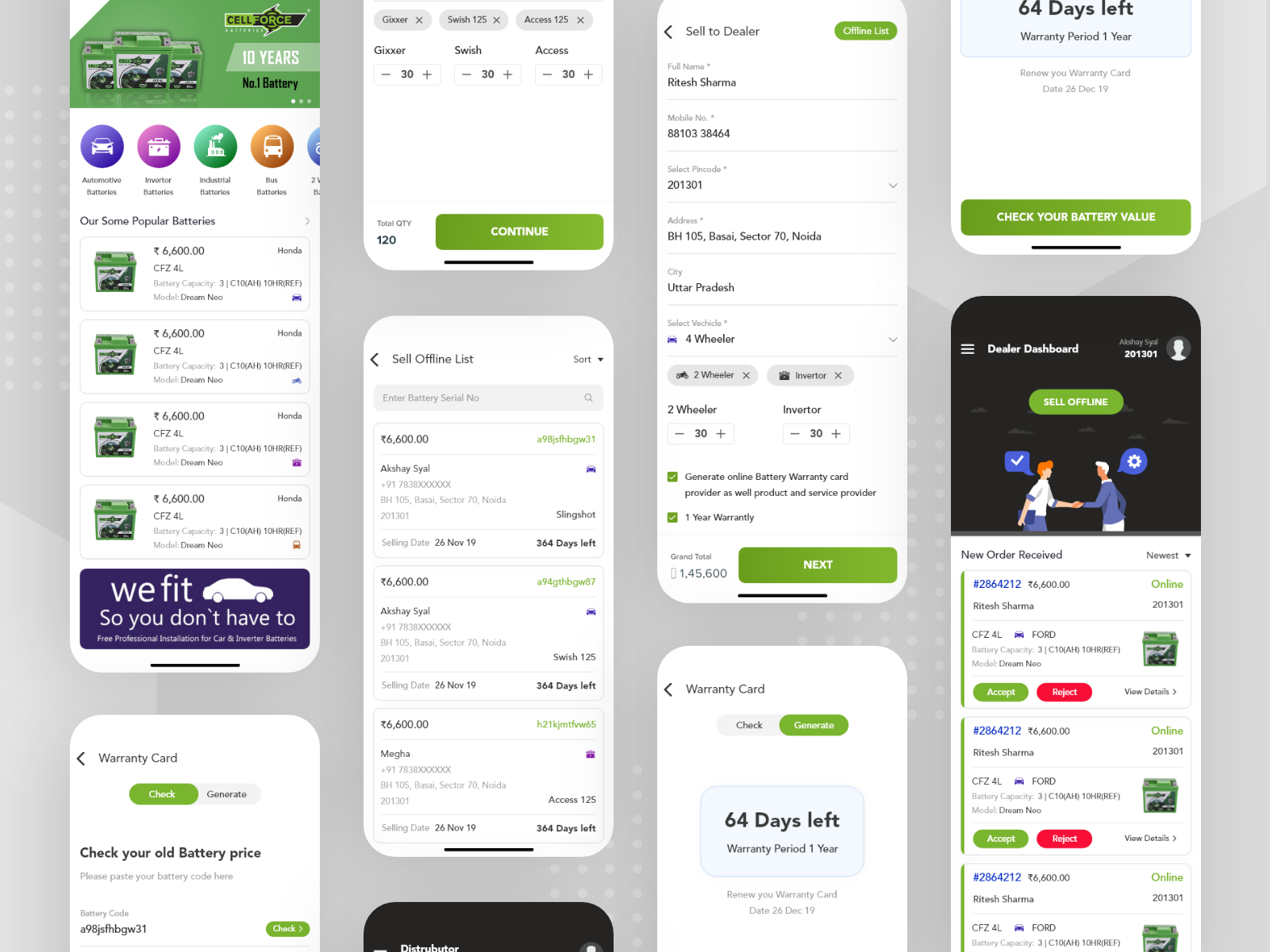The image displays a screenshot of an application interface set against a gray background, with a series of mobile screens arranged in vertical columns. Each mobile screen displays different items predominantly related to battery packs. One screen highlights a variety of battery packs, labeled as "Cell Force," noting "10 years, number one battery," and includes specifications like "6,600" and "CFCZ4L." Another screen features a slogan, "WeFit, so you don't have to," alongside additional battery pack images. Text such as "selling date" and "sell offline list" is visible at the top of these screens.

On the right-hand side of the image, there's a dealer dashboard interface with an option to "Sell Offline." This section also includes an icon of two people shaking hands: one person has a blue checkmark on a blue background, and the other has a settings gear icon also on a blue background. Listings under the dashboard include "Retail Sharma," with indicators like "online 201" and "301," as well as details about a warranty card stating "64 days left" of a "warranty period of one year."